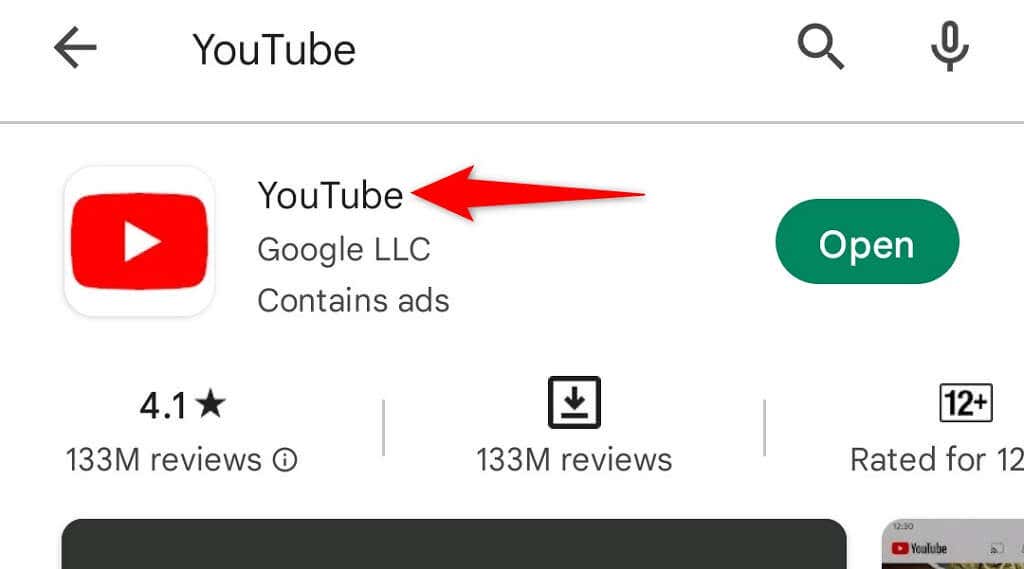This screenshot shows the YouTube app on a mobile device interface. At the top-left corner, there's a black left-facing arrow. To its right, the YouTube logo is displayed with "YouTube" in a combination of capital and lowercase letters ("Y" and "T" are capitalized). On the top-right corner, there's a search icon followed by a microphone icon.

Below this header, there's a thin horizontal gray line extending across the screen. Just beneath this line, on the left, there's a prominent red button featuring a white arrow in a white diamond shape, indicating a YouTube branding element. Next to this button, it says "YouTube Google LLC" followed by the note "contains ads." 

Adjacent to the YouTube title, another red arrow is facing left. To its right, there's a green button labeled "OPEN" in large white font.

Underneath, on the left, it shows "4.1 stars" followed by "133M reviews." In the center, the "133M reviews" text is repeated, accompanied by a down arrow enclosed in a box. On the right-hand side, there's a box stating "12+" with the additional text "Rated for 12" below it.

At the bottom-left of the screenshot, a black bar stretches across three-quarters of the screen. On the bottom-right corner, a small gray bar contains the word "YouTube" in black text, preceded by a red box with a white arrow indicating YouTube's logo. The lower part of the image is cut off, obscuring some information.

The overall layout of the image provides details of the YouTube app, including rating information, review summary, and app interface elements.